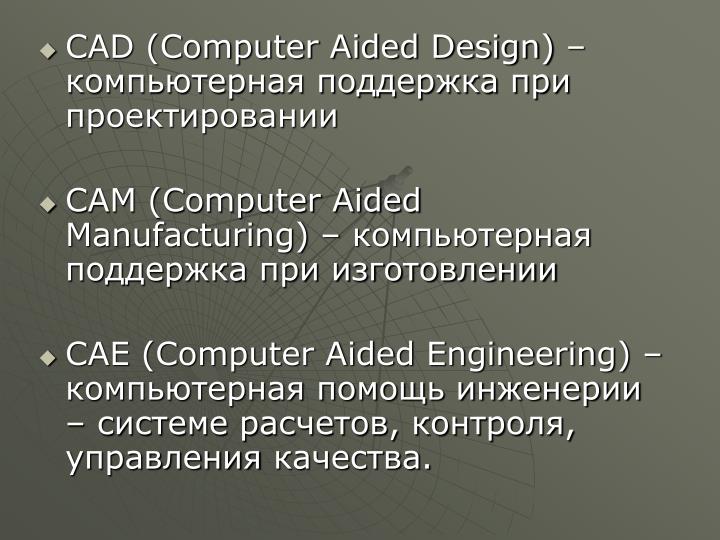This PowerPoint slide has a gray background with a faint image of a large satellite dish, specifically a radio telescope, pointing up and to the right. The dish has a grid pattern and four metal rods converging at a point. Overlaying the background are three diamond-shaped bullet points with black shadowing. Each bullet point features text in both English and Russian, written in white letters with black shadowing.

1. **CAD** (Computer Aided Design) — followed by Russian text.
2. **CAM** (Computer Aided Manufacturing) — followed by Russian text.
3. **CAE** (Computer Aided Engineering) — followed by Russian text.

The text is arranged in three lines for the first two points and four lines for the third, making the information clear and structured. This detailed slide serves as an informative graphic on computer-aided technologies.